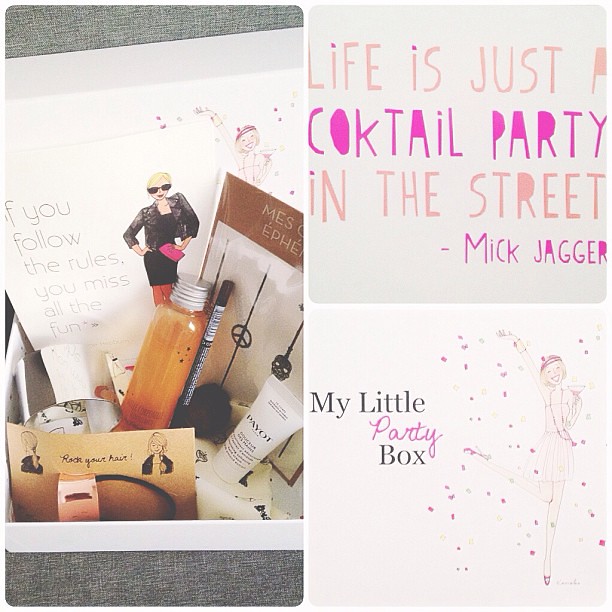This image is a meticulously arranged collage that combines both photographs and illustrations, presenting a vivid and stylish composition. On the left side, a photograph captures a top-down view into an open gray box filled with various beauty and grooming items, such as lotions, a thin eye pencil, a white tube labeled "P-A-Y-O-T," and an amber-colored liquid in a bottle. The box's inner lid features a card with an illustration of a blonde woman in a black dress, a pink handbag, and shades, accompanied by the text: "If you follow the rules, you'll miss all the fun." Another card in the box bears the slogan "Rock your hair" and includes drawings of two people with ponytails.

To the right are two vertically stacked squares. The upper square has a gray background with light peach and pink painted text that reads: "Life is just a cocktail party in the street," followed by the signature "Mick Jagger." The words "cocktail party" are prominently illustrated with a misspelling as "C-O-K-T-A-I-L." The lower square showcases a light pink background with an illustration of a joyous woman holding a cocktail while throwing confetti. The accompanying text reads, "My Little Party Box," with "my little" and "box" in gray, and "party" in pink. The overall style of the montage reflects a blend of photographic realism and illustrative graphic design, celebrating a lively and playful theme.